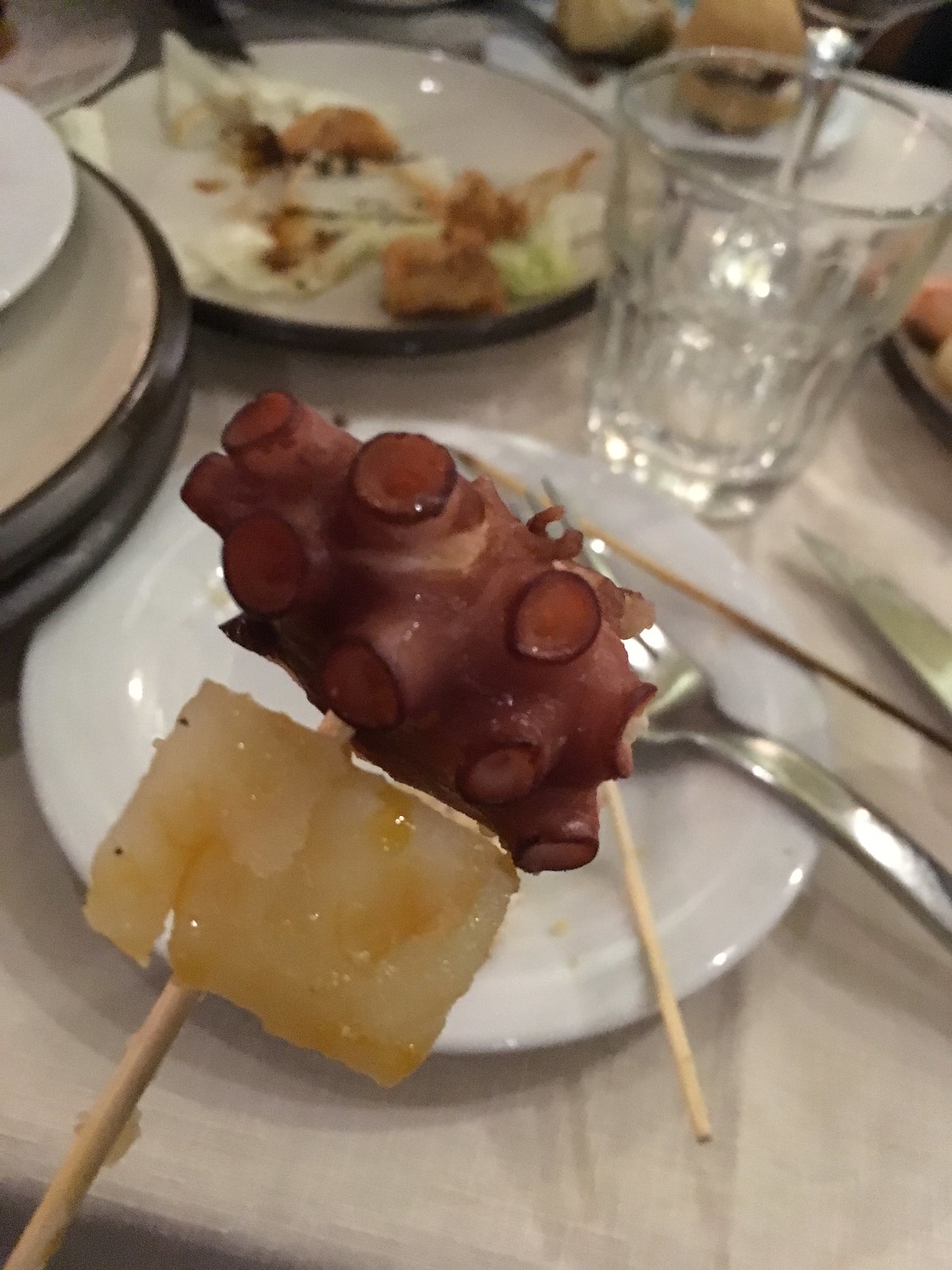This close-up image taken inside a restaurant showcases a sophisticated table setting with a white tablecloth. Dominating the foreground is a brownish skewer with two types of seafood at its tip. The top-most piece is an unmistakable octopus tentacle, characterized by its reddish-pink hue and distinctive black-ringed suction cups. Below it, sits a rectangular-shaped piece of seafood, likely a scallop, sporting a white and yellowish tint. A circular white plate featuring a silver fork and knife provides the backdrop, accompanied by two thin, empty skewers. To the upper half of the image, a large bowl containing greens and possibly bread sits next to what appears to be a plate of sliders. A clear drinking glass and a stack of plates, including a white, a silver, and a black one, add to the detailed, elegant table arrangement.